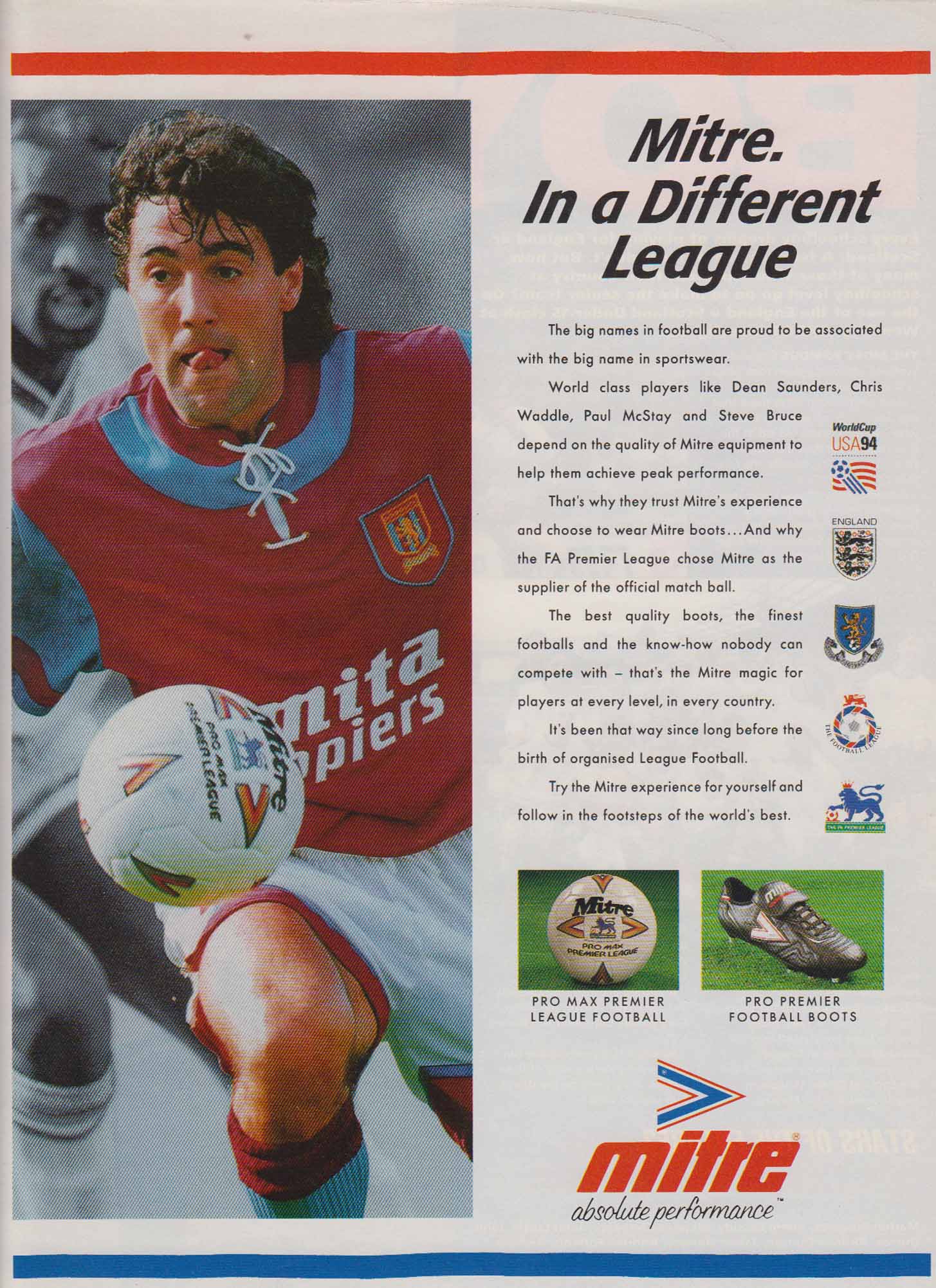The image is a detailed soccer poster, primarily on a white background with bold black text. A striking red bar stretches horizontally across the top, while a complementary blue bar runs along the bottom. Dominating the left half of the poster is a photo of two soccer players in action. The player in focus is vividly colored, wearing a red and blue shirt with a circular white-laced collar, white shorts with red stripes at the bottom, and white socks featuring red knee stripes. This player appears to be mid-kick, with his left knee raised, ready to strike the soccer ball marked with the word "Mitre." In contrast, the second player is shown in black and white, leaning to the left with thick curly hair and his tongue sticking out.

Adjacent to the photo, on the right side, the main text reads "Mitre" and "In a Different League." Beneath this heading, six paragraphs extol the virtues of the brand, mentioning that big names in football are proud to be associated with Mitre sportswear. The right side of the poster is further adorned with multiple logos, including the World Cup USA 94 England logo, an Alliance logo, and a Mitre soccer ball icon. Just below these, accompanying images highlight "Pro Premier Football Boots" and another Mitre logo. The poster concludes with the slogan "Mitre: Absolute Performance" at the bottom.